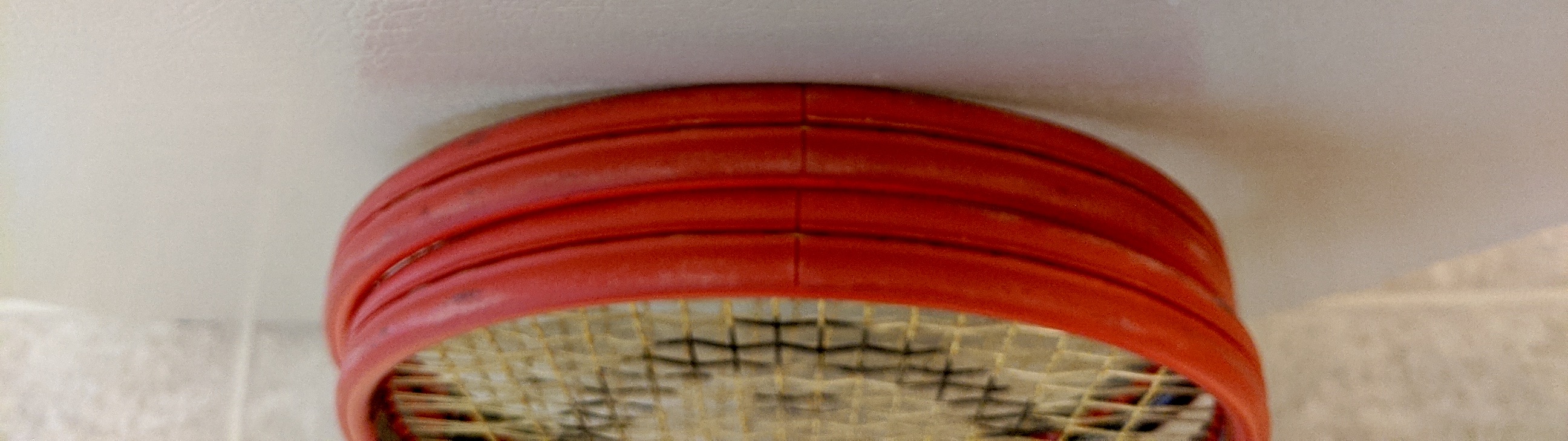The image depicts a pair of bright red tennis rackets stacked on top of each other on what appears to be a gray table, which is situated against a wall featuring white, textured subway tiles. The rackets have a gradient design incorporating white and yellow hues. There is a noticeable, thick layer of red around the edge of the rackets. The netting, which is a mix of beige and brown, is visible through the strings and appears sturdy. The rackets also feature a black logo designating their brand on the frame where the strings are attached. The setup of the image gives it a somewhat cropped and upside-down appearance, with the upper portion of the rackets distinctly visible, highlighting the circular design on them.